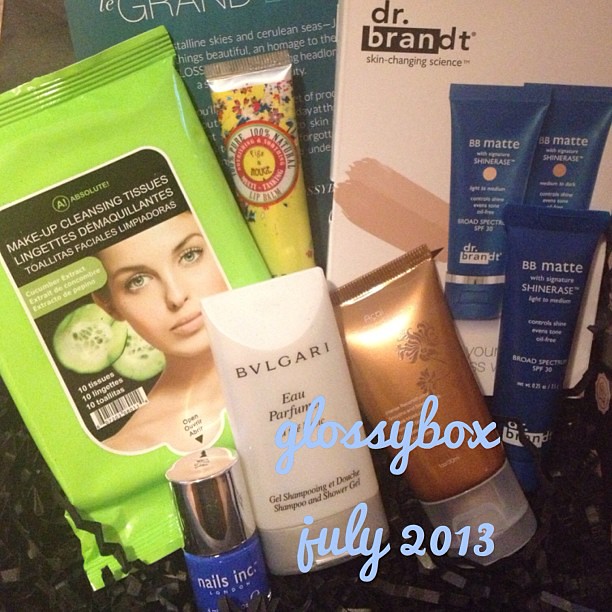The photograph displays an array of skincare and beauty products arranged on a backdrop of crumpled, thinly cut black paper streamers. In the bottom right corner, blue cursive text reads "Glossy Box July 2013." Prominently featured is a lime green package of makeup cleansing tissues with an image of a Caucasian woman and cucumbers. Nearby is a light white bottle labeled Bvlgari, a bronze or gold squeeze bottle, and a smaller blue squeeze bottle marked BB Matte Shine Erase. Behind these items is a large white box labeled "Dr. Brandt Skin Changing Science," adorned with images of blue tubes. The central background showcases a yellow bottle with a silver top and a white circle inscribed with floral designs. Additionally, a teal blue package partially obscured by other items is visible. This meticulously arranged assortment highlights the diversity and elegance of the beauty and skincare products showcased in the Glossy Box of July 2013.